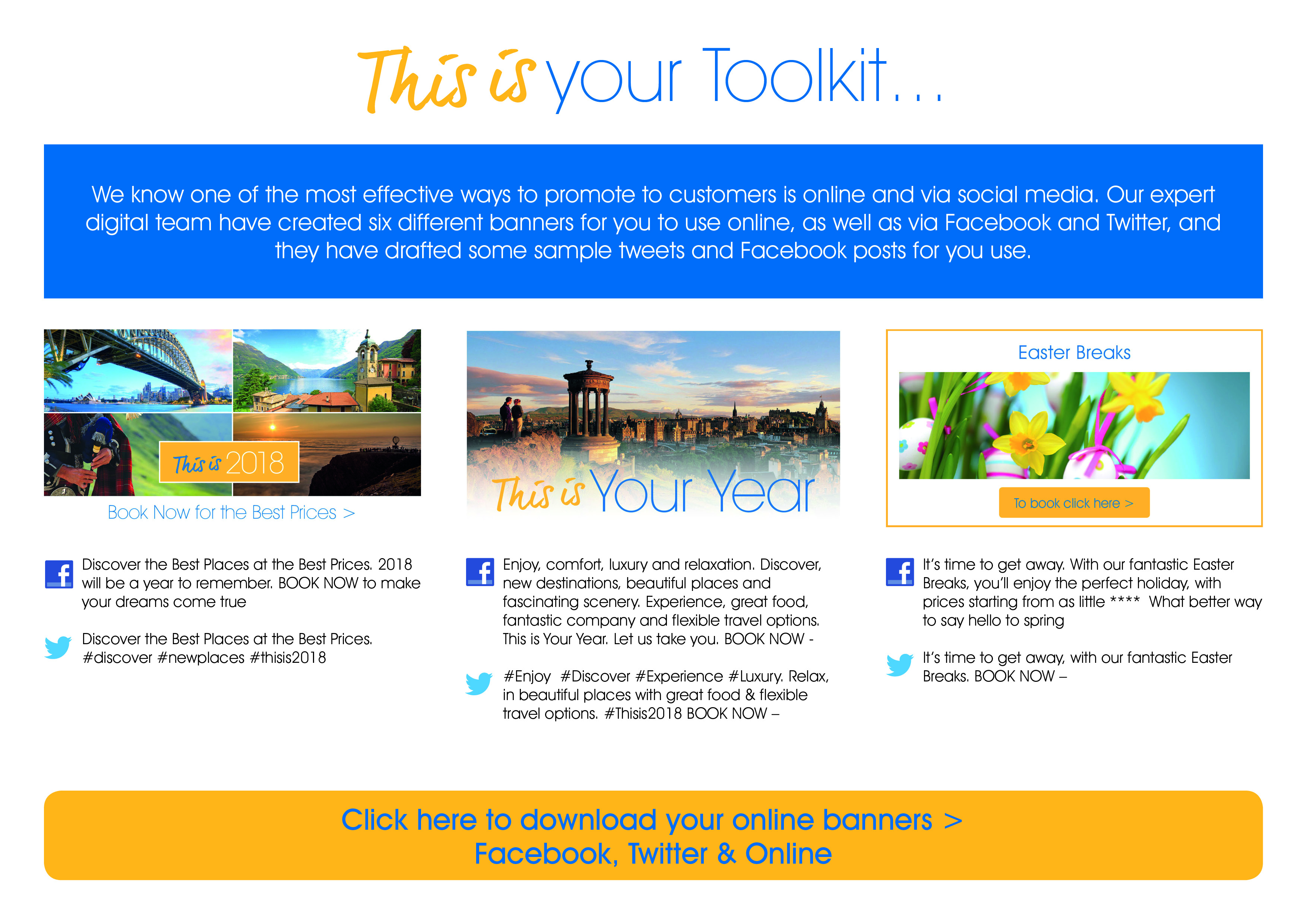This is a detailed descriptive caption for the provided image:

The screenshot displays an advertisement designed to promote a travel service. At the top, a sleek white bar contains the text "This is" written in elegant cursive yellow font, followed by "Your Toolkit..." in bold blue font. Immediately below, a dark blue bar features white text explaining the advertisement's purpose: "We know one of the most effective ways to promote to customers is online and via social media. Our expert digital team has created six different banners for you to use online, as well as via Facebook and Twitter, and they have drafted some simple tweets and Facebook posts for you to use."

Directly beneath this explanatory section, three visually engaging advertisements are displayed in a horizontal row. On the left, there is a postcard-style graphic showcasing four stunning landscapes, each depicting a unique travel destination. Overlaid on the postcard is an eye-catching orange rectangle with the bold text "This is 2018" in white. Below this, in large blue font, the prompt "Book now for the best prices" urges immediate action.

Further down in the right corner, a Facebook logo is accompanied by a promotional message that reads, "Discover the best places at the best prices. 2018 will be a year to remember. Book now to make your dreams come true." Similarly, a Twitter symbol is paired with a tweet-ready caption: "Discover the best places for the best prices. #discover #newplaces #thisis2018."

This advertisement leverages visually appealing graphics and compelling text to encourage potential customers to engage with their travel services via social media platforms.